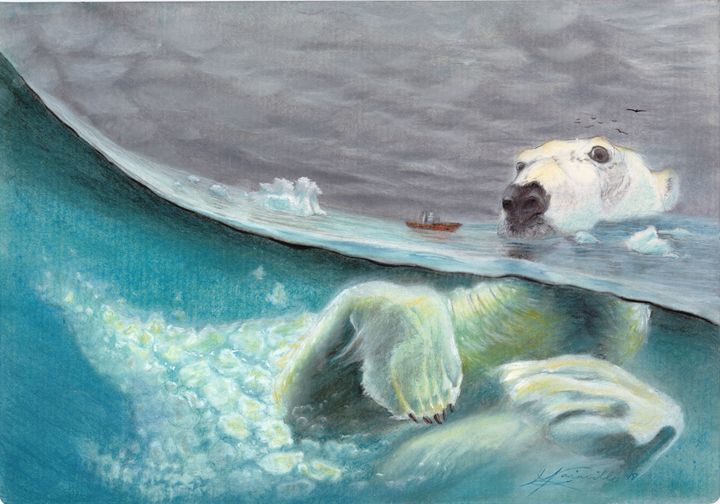This rectangular, landscape-oriented color painting, approximately five inches wide by four inches high, appears to be created with colored pencils or a similar medium. The artwork is divided into two sections: above and below the water surface. The upper half features a dark gray, cloud-filled sky adorned with a few dark birds in the top right corner. Below the sky is a blue and white ocean surface, populated with several floating ice structures primarily in the upper left region of the image. 

Dominating the right side of the horizon is the large head of a polar bear emerging from the water. Next to it, a small brown boat sits in stark contrast, nearly the size of the bear's nose, emphasizing its immense scale. 

The lower section provides an underwater view of the polar bear's body, where the neck and front paws are clearly visible, while the rest of its body fades into a blend of blue water and white bubbles. A subtle S-curve wave traverses from the top left to the bottom right, creating a dynamic diagonal across the center. In the lower right-hand corner, an illegible blue signature marks the artist's presence.